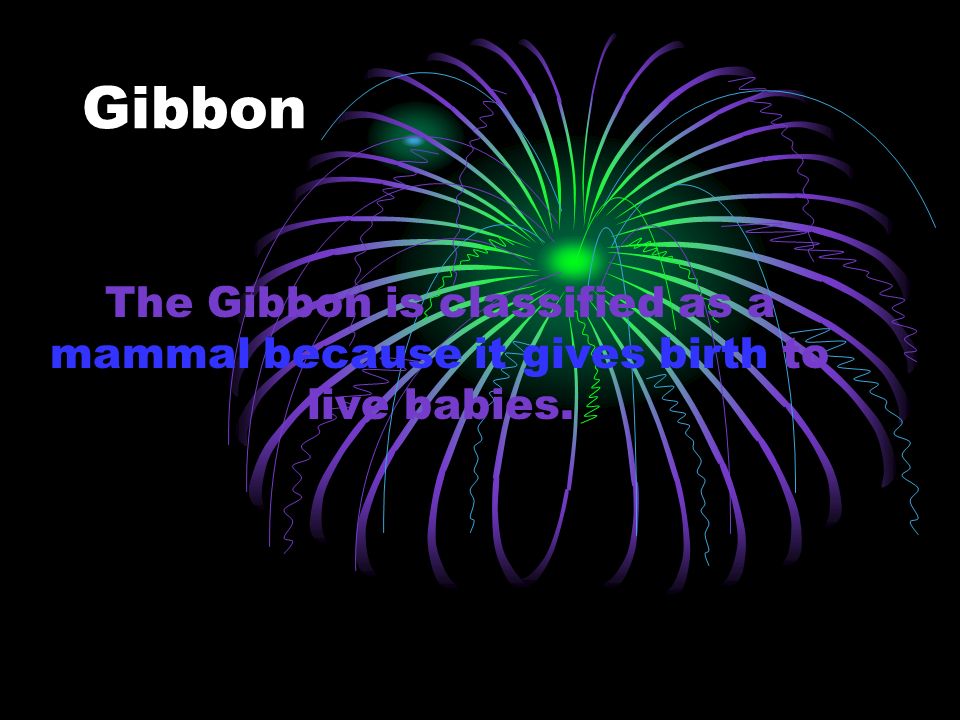The image appears to be a PowerPoint slide or a Google slide with a black background. Central to the slide, slightly offset to the right, is a vibrant graphic resembling a firework with a green center and purple tendrils radiating outward in a manner akin to a mushroom cloud. Overlaid on this graphic is the text "The given is classified as a mammal because it gives birth to live babies," written in blue and purple letters, with the phrases "mammal because it gives birth" in blue. The word "given," in white text, is positioned in the upper left corner of the slide, separate from the rest of the text. The overall imagery and text styling suggest an academic presentation, with the colorful graphic adding visual interest but not directly related to the textual content.